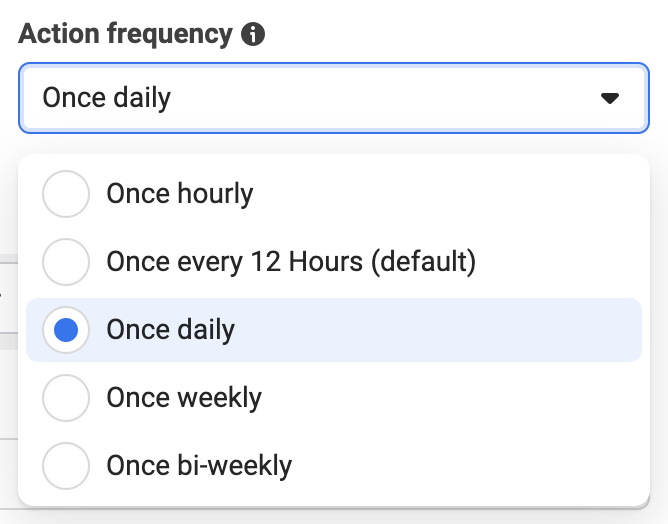The image showcases a user interface for configuring action frequency settings. In the top left corner, the text "Action Frequency" is prominently displayed in black font. Adjacent to this text, on the right, is a black circle containing a white letter "I," indicating informational content.

Directly below this title is a rectangular selection box outlined in blue, which gradually transitions to a lighter blue shade towards the center. On the left end of this box, the phrase "Once Daily" is displayed, while on the far right, a black downward-facing arrow suggests the presence of a dropdown menu.

Further below, within a larger, similarly bordered rectangular area with a blue outline, are five circular radio buttons aligned on the left. Each button is accompanied by descriptive text:

1. "Once Hourly" next to the first circle,
2. "Once Every 12 Hours, default" next to the second circle,
3. The third circle, which is filled with a blue dot indicating it is selected, labeled "Once Daily" and highlighted with a blue background,
4. "Once Weekly" beside the fourth circle,
5. "Once Biweekly" next to the fifth circle.

The background of this section is a subtle whitish-gray gradient, providing a clean contrast to the text and buttons.